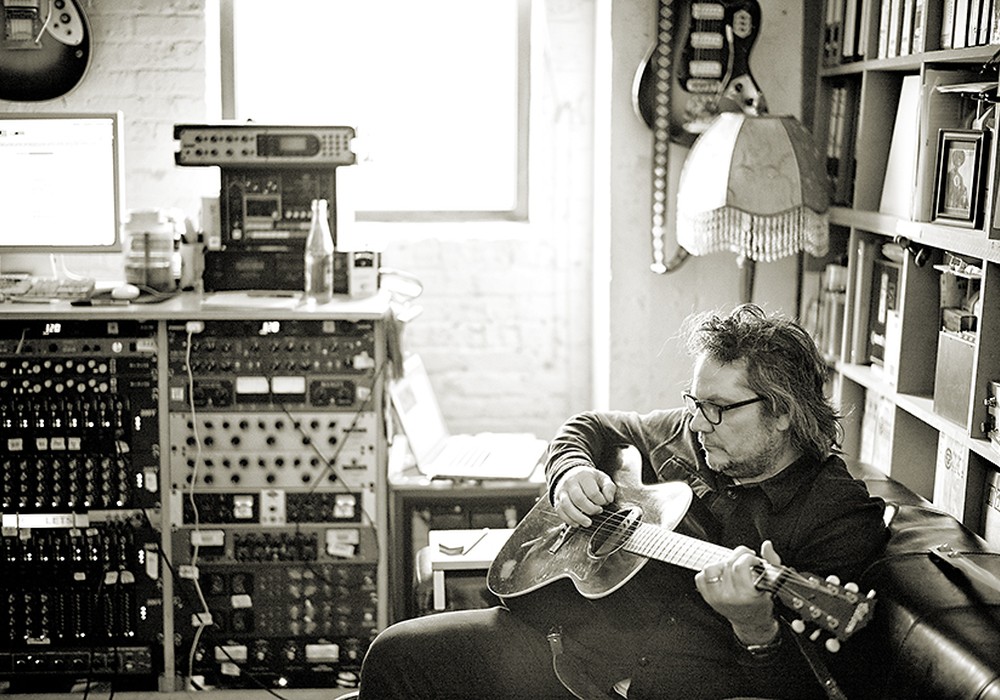In this black-and-white photograph, an older Caucasian man, possibly in his fifties, is seated on a black leather couch, absorbed in playing a worn, aged guitar. His appearance is unkempt, with long hair cascading past his collar, a stubbly beard extending just below his chin, and he wears black-framed glasses. Dressed in a long-sleeve black shirt and black pants, he also sports a wedding ring and a watch. The setting appears to be a recording studio, with a variety of musical and electronic equipment surrounding him. To his sides, electric guitars are mounted on the cream-colored brick walls; one guitar is left and another to the right, near a window that lets in daylight. Behind him, a bookshelf brims with books and framed photographs. A fringed lamp stands out among the backdrop of the organized clutter. In front of him lies a bank of sound equipment with numerous knobs, buttons, and hanging cords, along with an open laptop and a water bottle. This detailed environment suggests a space dedicated to music creation and arrangement.